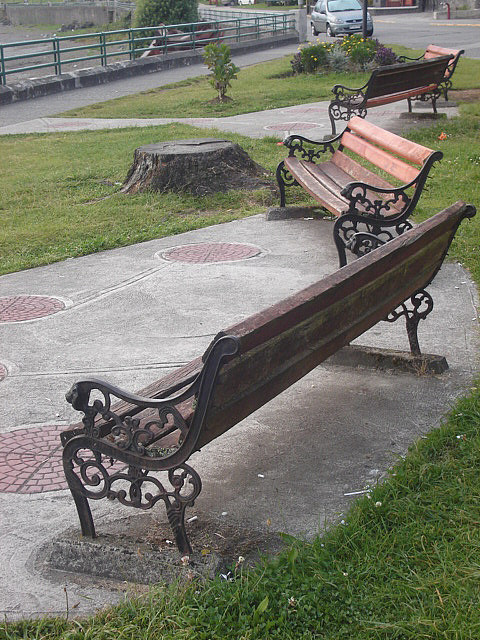In this photograph, we see a tranquil seating area featuring four park benches laid out side by side. The benches, constructed with wooden slats, exhibit a rustic reddish color on the seat and backrest. They rest on wrought iron armrests and legs, which are finished with a patina hue and anchored to concrete bases. Surrounding the benches is a concrete pad adorned with a red circular brick pattern interspersed with gray bricks, and the area is fringed with well-manicured, green grass. 

Central to the image is an aged tree stump, cut down long ago, positioned behind the benches. This setting appears to be a viewing area possibly overlooking a spillway or river, as indicated by metal railings that section off the area and suggest a sloping drop-off beyond sight. In the top left corner, metal handrails are visible, while in the top right corner, a road with a car driving by can be seen, adding to the serene yet active ambiance of the park. Additional elements include a manhole cover on the concrete pad and a small garden with flowers adding a touch of color and life to the scene.